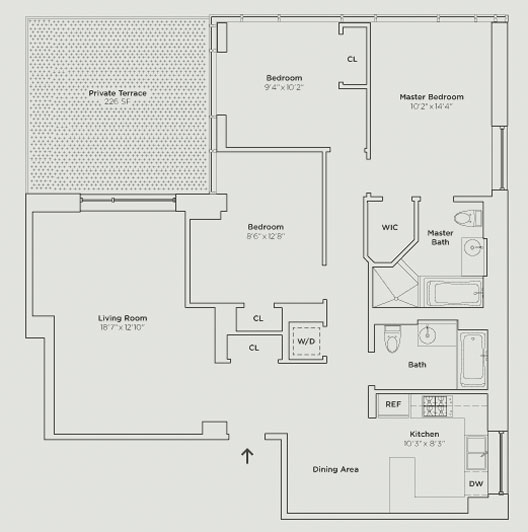This is a meticulously detailed floor plan of a single-story residence, showcasing a layout that is rectangular but nearly a perfect square, with a few cutouts on the left-hand side. The plan features a variety of spaces, including a private terrace distinguished by its hatch pattern, unlike the unshaded walls throughout the rest of the house. 

At the bottom of the page, the kitchen and dining room are prominently positioned, forming the front part of the layout. On the top right corner of the page, the three bedrooms are thoughtfully arranged—a standard bedroom, a master bedroom, and another bedroom are all located in this quadrant. The master bedroom is accompanied by a master bath for added luxury, while a secondary bath is conveniently placed off the kitchen. Additionally, a spacious living room links these areas, providing a central communal space.

Thank you for taking the time to explore this floor plan.